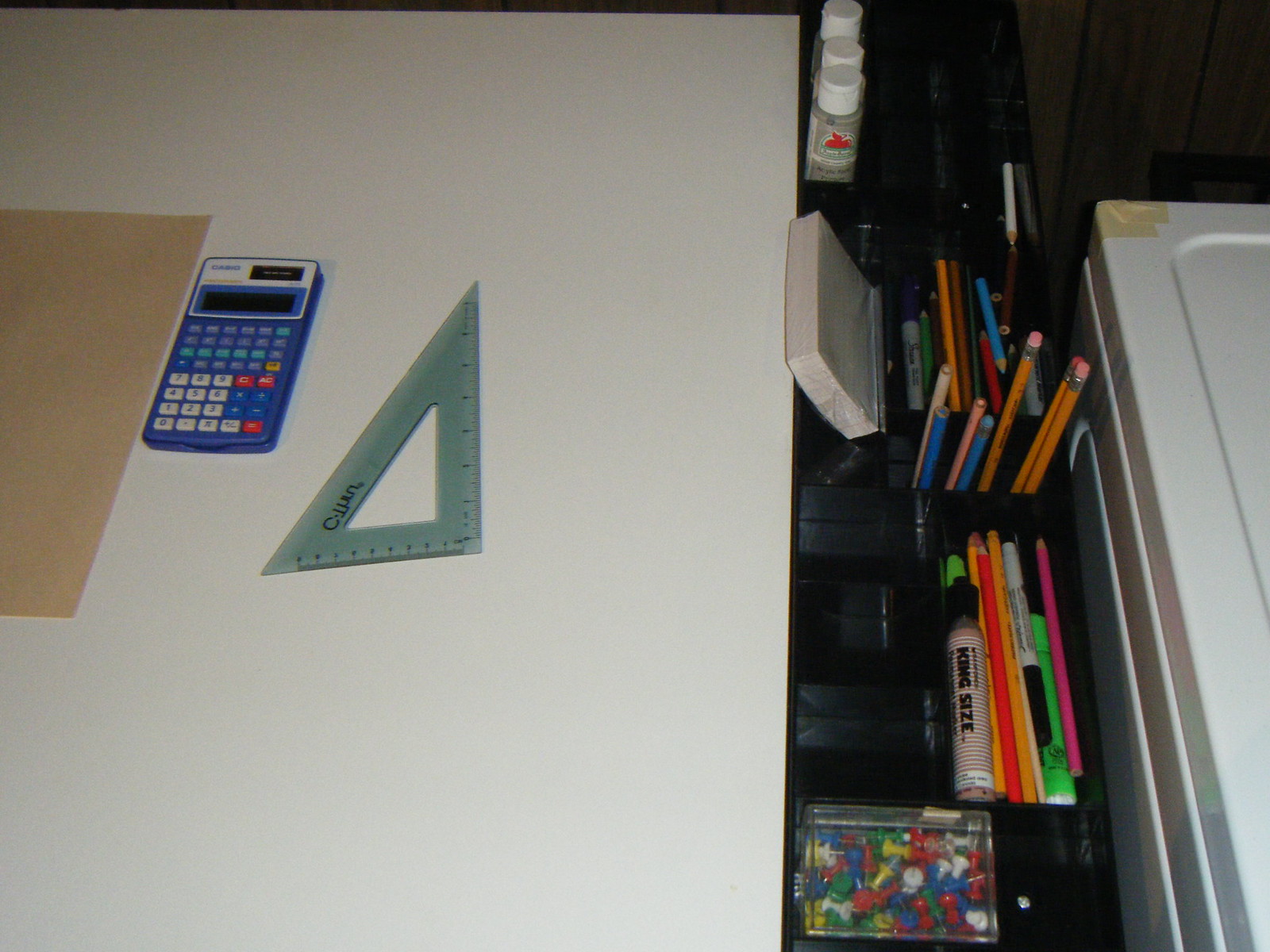The image showcases a neatly organized desk area, viewed from a slightly elevated angle. The setting appears to be indoors, characterized by a muted, gray background with minimal lighting. In the upper right-hand corner, a bulletin board or some similar structure is partially visible, enhancing the organized atmosphere.

Prominently displayed on the desk is a white surface, which could either be a poster board or a table. On this surface, various objects are meticulously arranged. There's a brown piece of paper extending towards the left, cropped off by the image's frame. Next to it sits a blue calculator, slightly more advanced than a basic model, though its specific functions are not discernible from the image.

A white container with black masking tape around its rounded edges is situated nearby. In addition, several black trays are neatly filled with an array of office and school supplies, including pencils, colored pencils, note cards, markers, Sharpies, and thumbtacks—all systematically organized within the compartments.

Also noteworthy is a triangular ruler, designed for precise tracing and outlining, adding to the overall impression of an efficient, well-equipped workspace.